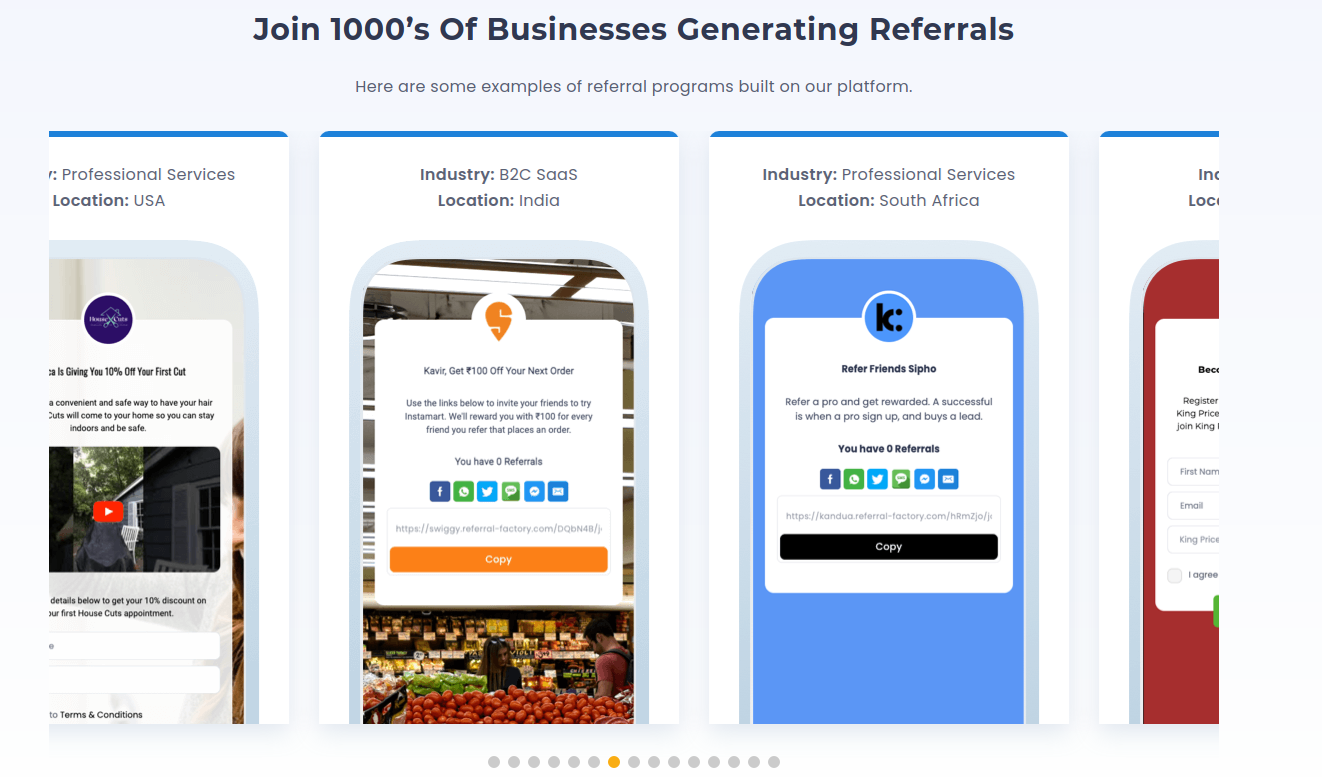The image features a blue rectangle with darker blue text that reads "Join thousands of businesses generating referrals." Beneath this prominent slogan is smaller text that is difficult to read. Below the main blue rectangle, there are a series of three white rectangles, each with a blue line atop, showcasing different phone screens.

1. **First Phone:** The screen is partially cut off on the left side. It contains a video thumbnail with a red rectangle in the middle and a right-pointing arrow, indicative of a play button. There is some unreadable text below the video thumbnail.

2. **Second Phone:** The top part of the phone screen displays some text. Below this, the screen shows a white circle with an unusual 'S' symbol in it, resembling a logo. This is followed by a white rectangle containing text and a series of various symbols that appear to be social media icons, although not all are clearly identifiable. An orange rectangle with text is also visible.

3. **Third Phone:** The screen has text at the top, followed by a design of a blue phone with a darker blue interior. A blue circle outlined in white features a 'K' and a colon. Below this is a white rectangle with more text, additional icons that might be social media icons, and more text. The sequence ends with a black rectangle containing a single word.

The fourth and partially visible phone screen has a blue exterior with a red interior, and a portion of a white rectangle can be seen.